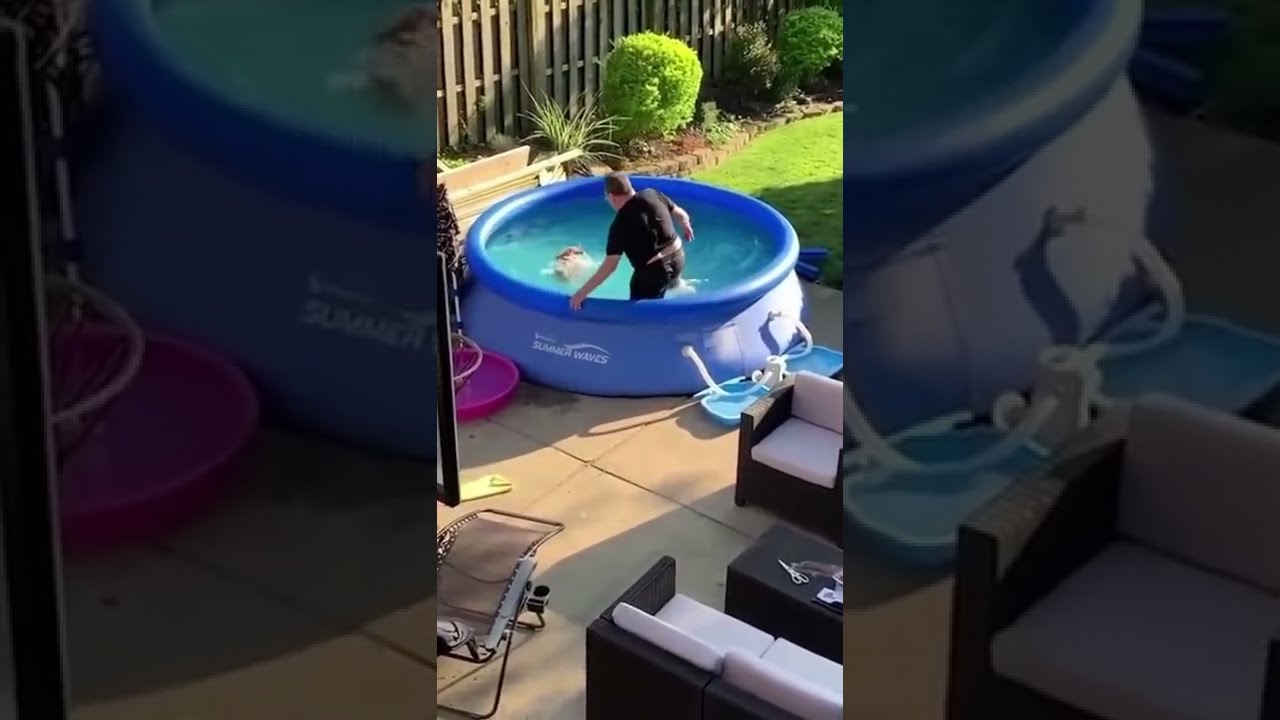In a neatly maintained backyard with lush green grass and a wooden tall fence adorned with shrubs, a large man, possibly in his 40s, stands in a blue, inflatable swimming pool marked with the logo "Summer Waves." The pool is approximately two feet deep, causing the water to reach the top of his thighs. The man is dressed in a wet black t-shirt and black bottoms, standing on a cement patio adjacent to the grass. He appears to be looking at a brown object in the water, possibly a small animal like a cat or dog, though it's hard to discern clearly.

Next to the inflatable pool, there is a smaller pink kiddie pool. The patio is furnished with a sophisticated outdoor seating set, featuring black wooden furniture with white cushions, and a black coffee table that holds a pair of silver scissors. Additionally, a zero-gravity lawn chair is placed nearby. The patio's flooring consists of large square sections, enhancing its modern aesthetic. Some blue objects are used to weigh down a pole with a handle attached to the pool. In the background, an enlarged and slightly lightened version of the main image is used, creating an artistic layered effect.